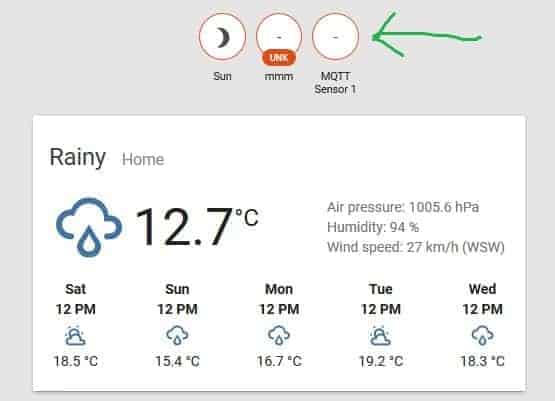This detailed caption describes an image of a weather application interface with a grey background. At the top center, there are three circles with reddish-orange outlines. The first circle on the left features an icon of a crescent moon facing left and the text "Sun," indicating Sunday. The middle circle contains a dash and the text "UNK" in white, surrounded by an oblong orange logo with the letters "MMM" beneath it. The circle on the right also displays a dash and is labeled "MQTT sensor 1" with a hand-drawn green arrow pointing towards it.

Below these circles, there is a white box with the bold word "rainy" and the text "home" in grey. Underneath, there is an image of a blue cloud with a single blue raindrop falling from it, accompanied by the bold text "12.7 degrees Celsius." The interface also provides additional weather details, including air pressure, humidity, and wind speed. Furthermore, it offers a forecast of predicted temperatures for Saturday, Sunday, Monday, Tuesday, and Wednesday, complete with icons representing different weather conditions such as sun and rain.